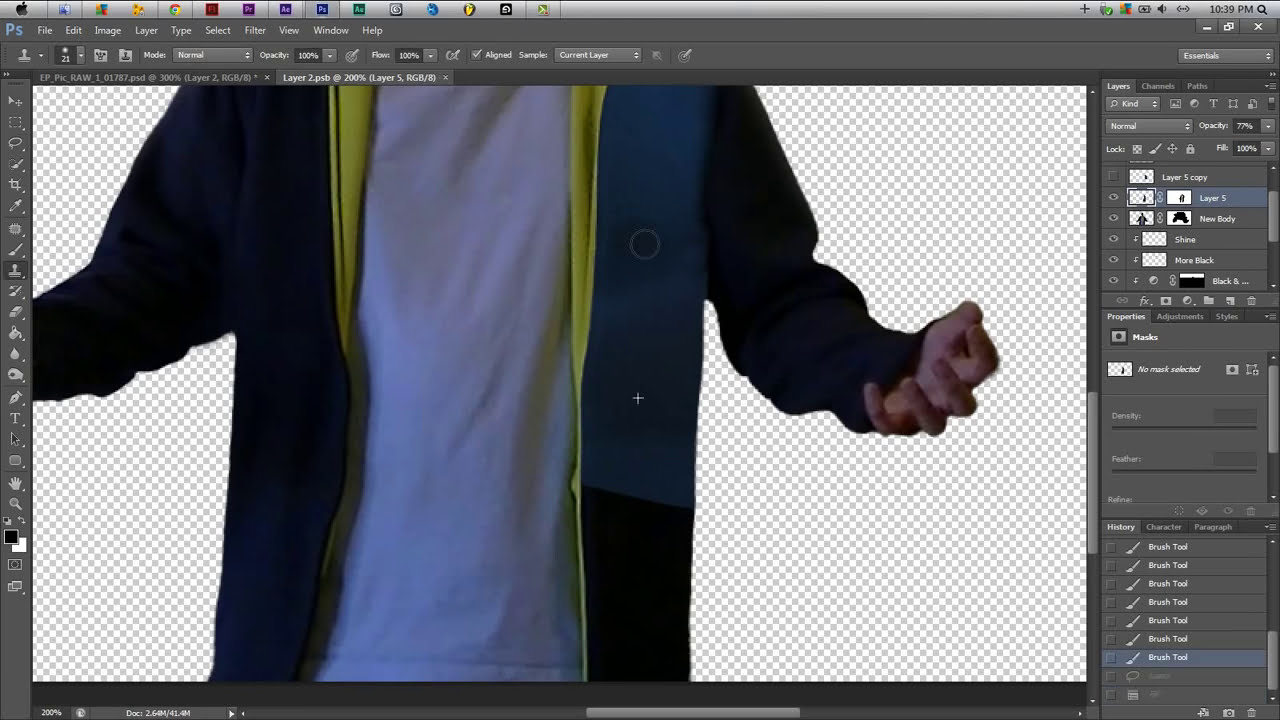This image appears to be a screenshot of Adobe Photoshop running on a Mac computer. Dominating the center of the screen is a zoomed-in section of a person's torso, showing a Caucasian individual wearing a blue jacket with a yellow interior and a white t-shirt underneath. The jacket features a darker blue section on the left side, which matches the color of the left sleeve, along with a black panel on the right-hand side. Surrounding the central image are various interface elements typical of Photoshop: a thin gray bar at the top displaying the Apple logo on the far left, along with app icons such as Finder, Windows, and Chrome, and the time on the right. Below this is the dark gray Photoshop interface, with menu options like File, Edit, and Image located at the top. On the left-hand side of the screen are editing tools such as the stamp, eraser, and fill tool, while the right-hand side is populated with various toolbars and properties panels for brush tools and other functionalities. The background of the canvas in the center is a transparent grid of small white and black squares. The entire scene is a detailed glimpse into a photo editing workflow on a Mac.